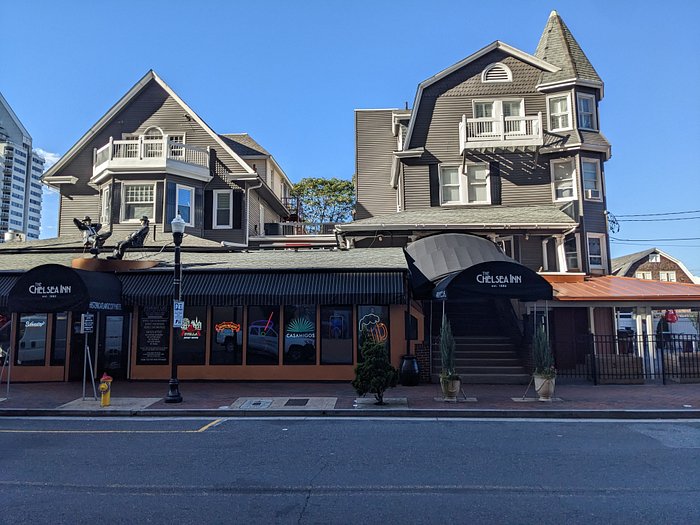The image captures a street view dominated by the Chelsea Inn, an older-style establishment that appears to integrate two historic gray houses with white trim and black shutters. The street-level business has two black and white striped awnings on both the left and right sides, reflecting a Broadway-style cover, perhaps for a valet service. In the forefront, the blacktop road features parking lines and a yellow fire hydrant on the left side. The scene is bathed in afternoon sunlight, casting shadows over the storefront and road, but illuminating the buildings above. The upper sections of the houses showcase white window woodwork and railings, along with balconies and a pointed tower on one structure. Neon signs, including one in the shape of a beer mug, are visible in the windows, while various plants adorn the exterior. Further in the background, additional city buildings are faintly visible, adding depth to this snapshot of urban life.